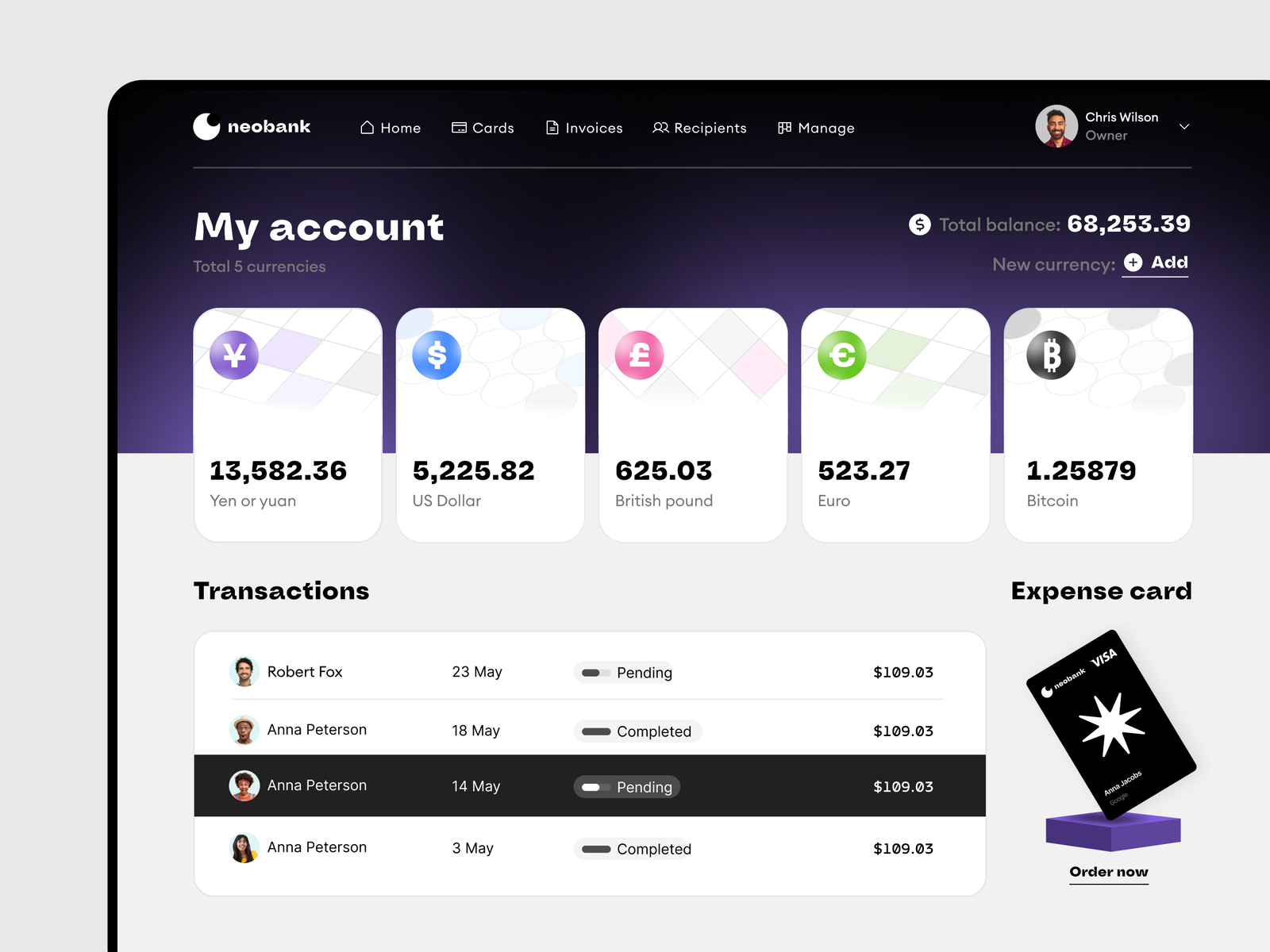The image is a detailed screenshot of a Neobank web page, depicting the account summary and transaction dashboard for a user named Chris Wilson, labeled as the owner. At the top of the page, the word "Neobank" is prominently displayed in white font on a black background. To the right, a small circular icon with a picture of a man's head and the name "Chris Wilson, owner" is visible. Below this header are various navigational tabs including Home (with a home icon), Cards (with a credit card icon), Invoices (with a paper icon), Recipients (with a heads icon), and Manage.

Beneath these tabs, on a purple background, there is a section labeled "My Account" with the note "Total five currencies" in white font. Five vertical rectangular blocks display different currency amounts: the first block shows a yin-yang symbol with its amount, followed by blocks for the US Dollar, British Pound, Euro, and Bitcoin. 

Further down, the "Transactions" section is highlighted over a gray background, featuring a white tab bar with entries displaying the name, icon, date, and amount. Additionally, there is a black card with a white star in the center, indicating a Visa card associated with Neobank, with an option for the customer to order the card.